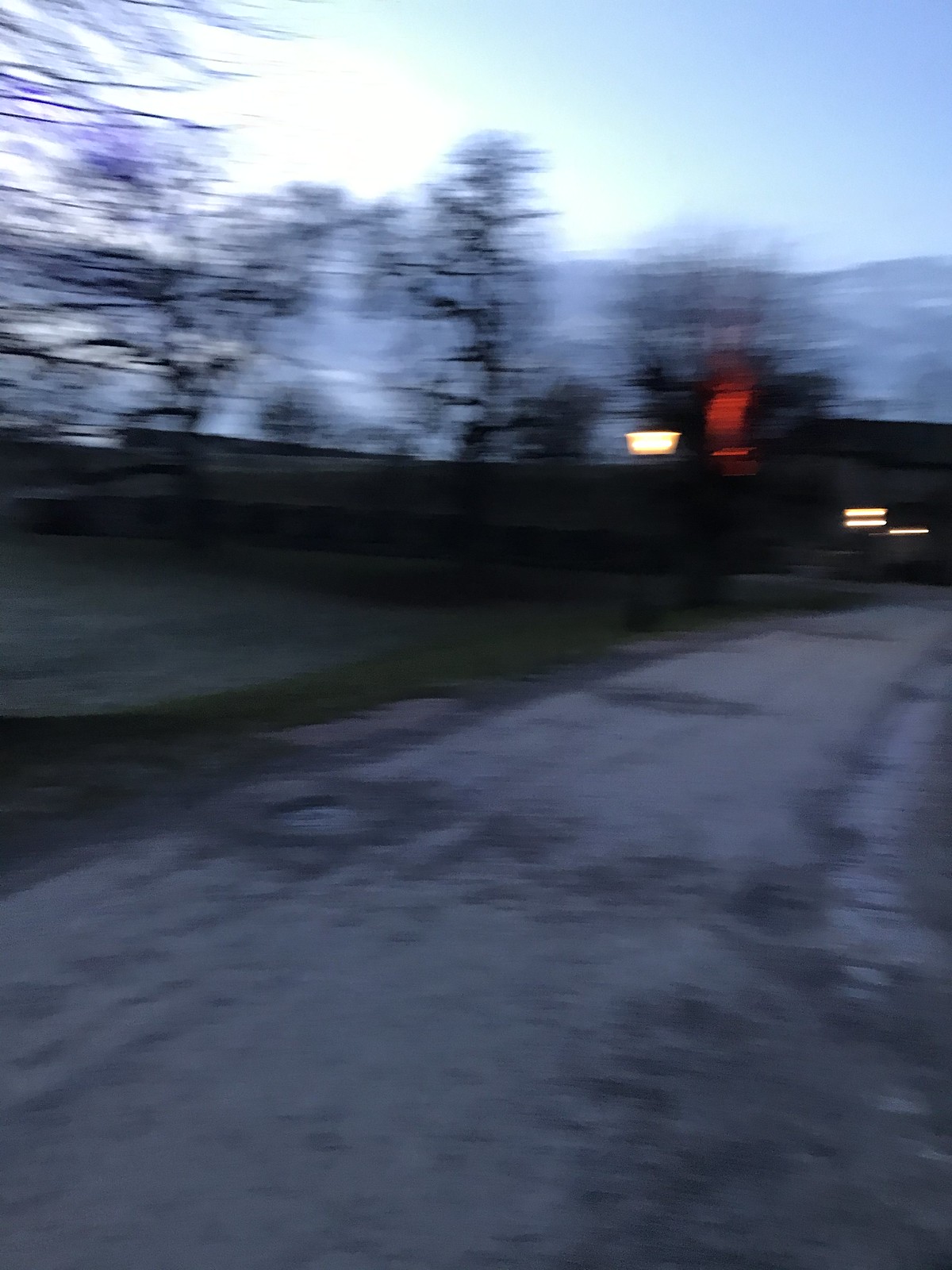In this image taken outdoors, the scene appears to be near sunset, indicated by the soft lighting. The sky is a clear blue with patches of white, perhaps from light clouds. In the background, leafless trees suggest that the season is either winter or early spring. These trees frame a long, concrete building extending from the right to the left of the frame, possibly a school, given its structure and faint illumination from a few lights inside. The foreground features what seems to be an old, worn asphalt road, giving the scene an almost rustic feel. The overall image is slightly blurry, adding a layer of charm to the serene yet cold environment.